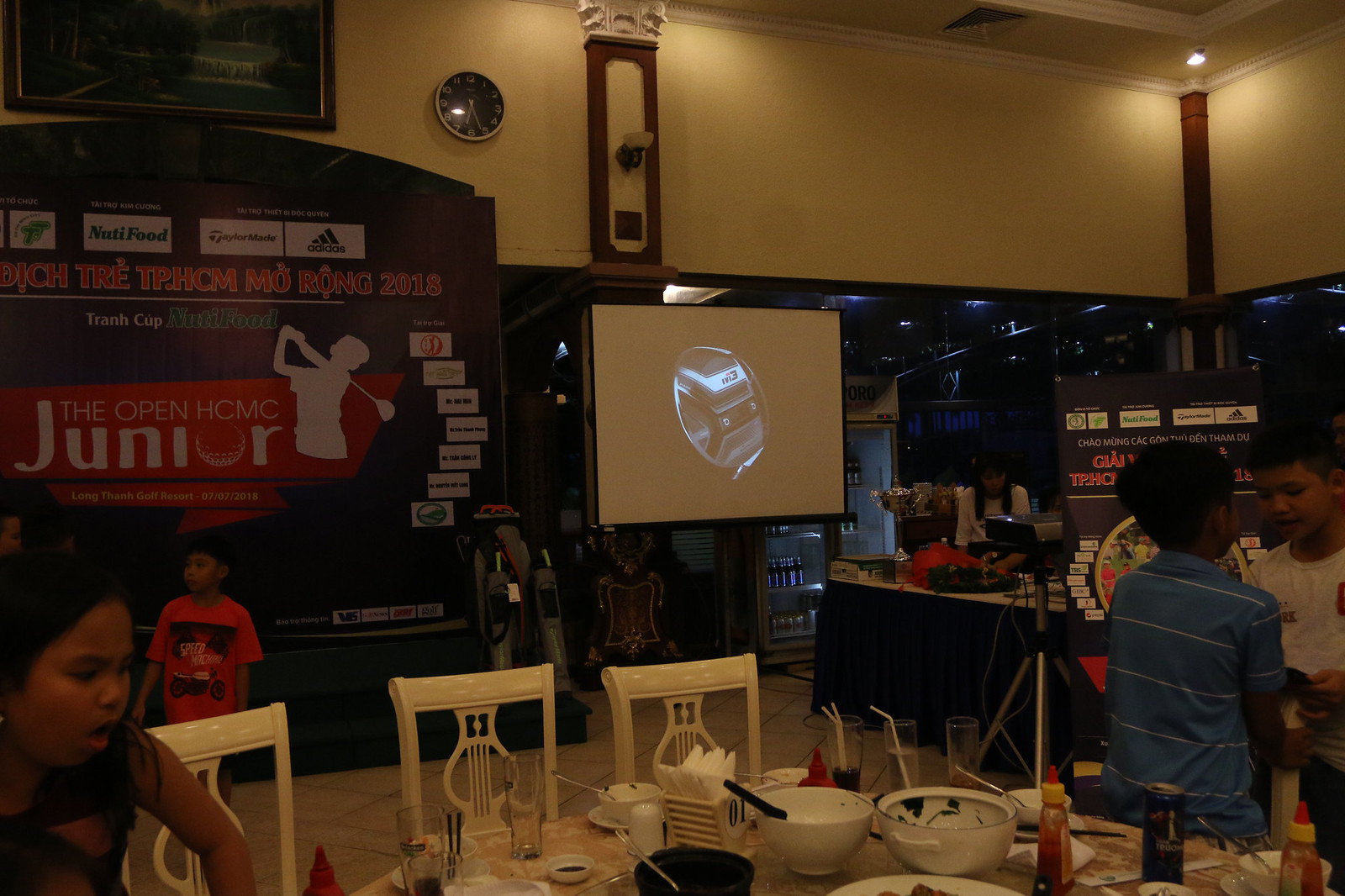In a dimly lit restaurant, large lights do little to illuminate the room, casting shadows that create a cozy atmosphere. This restaurant, with its Asian themed bowls—and unusually forks instead of chopsticks—and tall glasses with straws, appears to be hosting a special event. In the foreground, a table cluttered with various dishes and empty cups sits vacant, hinting at a recently concluded meal. A young girl sits quietly to the far left, while a boy in a red shirt walks by, and two boys in blue and white shirts chat nearby, their Southeast Asian features apparent. The event seems centered around golf as evidenced by the projector setup in the middle of the room, casting images onto a screen. On the left side of the screen, a detailed sign reads "The Open HCMC Junior Longthon Golf Resort 0707-2018" with a graphic of a person swinging a golf club, the text at the top in Vietnamese and sponsorship logos including Adidas. The entire setup suggests a golf benefit event for young participants, merging the ambiance of a traditional Asian restaurant with the excitement of a sports gathering.